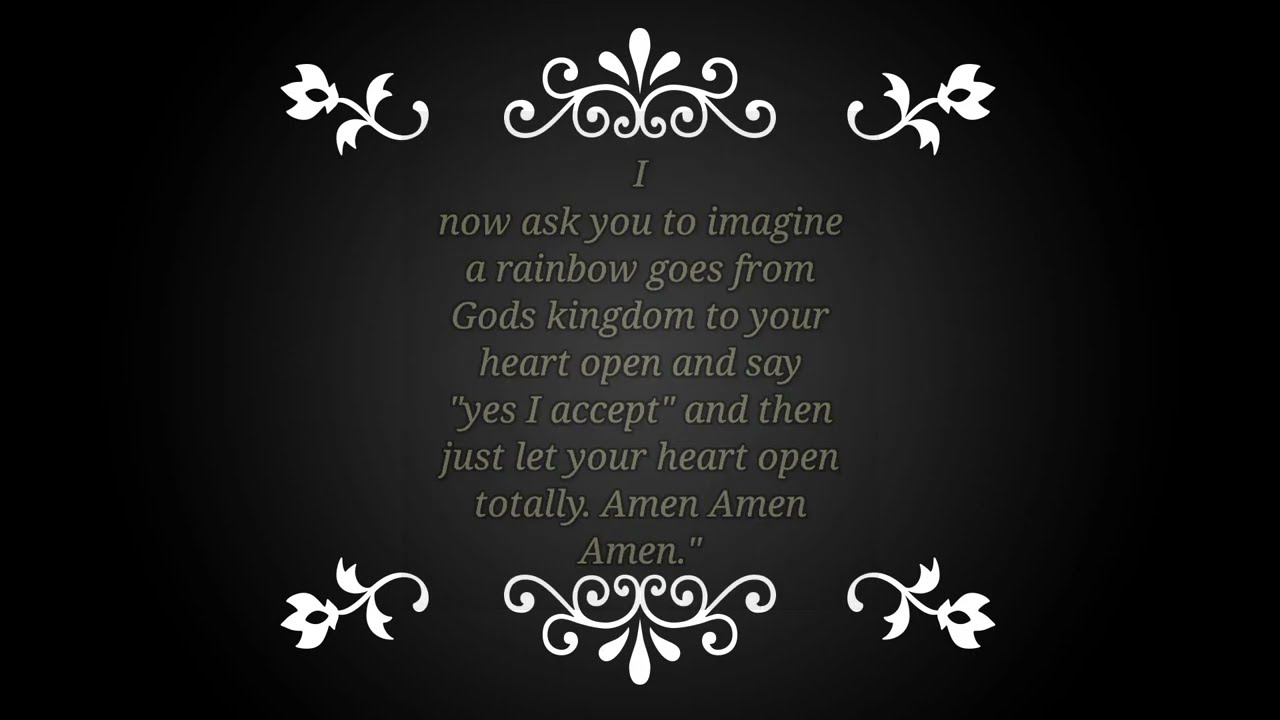The image centers around a prominent religious quote, with a completely black background that spans the entire canvas. Positioned directly in the middle is the textual focus, which reads: "I now ask you to imagine a rainbow goes from God's kingdom to your heart. Open and say, yes, I accept, and then just let your heart open totally. Amen, amen, amen." This text is displayed in varying shades of gray, contributing to a gray gradient effect that originates from the center and transitions to black on both sides. Surrounding the text are intricate floral designs—located in the upper left, lower left, upper right, and lower right corners of the image. Each design features curved flowers with stems and leaves that twist elegantly. Additionally, these floral motifs include curls and three prominent leaves at the center top and bottom of the text. The overall composition hints at a church poster or religious social media graphic, emphasizing serenity and spiritual openness.